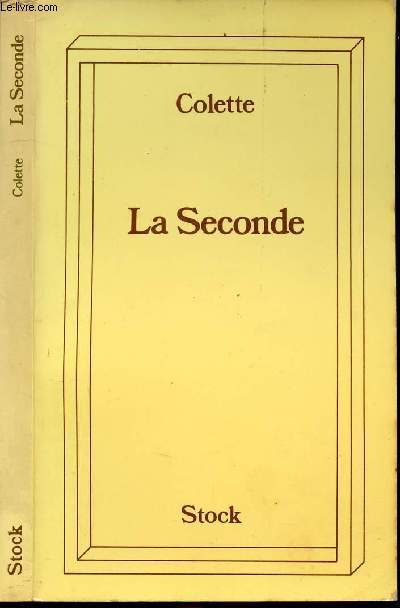The image depicts an old, possibly withered, book with a yellow or manila cover. Dominating the center is a minimalist 3D rectangle shape made up of roughly eight lines. Inside this rectangle, in a burgundy or dark brown font, it reads "Colette," followed by "La Seconde," and at the bottom, "Stock." On the left edge of the image, resembling the book's spine, the text "Stock, Colette, La Seconde" is written sideways. Additionally, at the top left corner, tiny text indicates photo attribution or a website, labeled as "LeLivre.com."